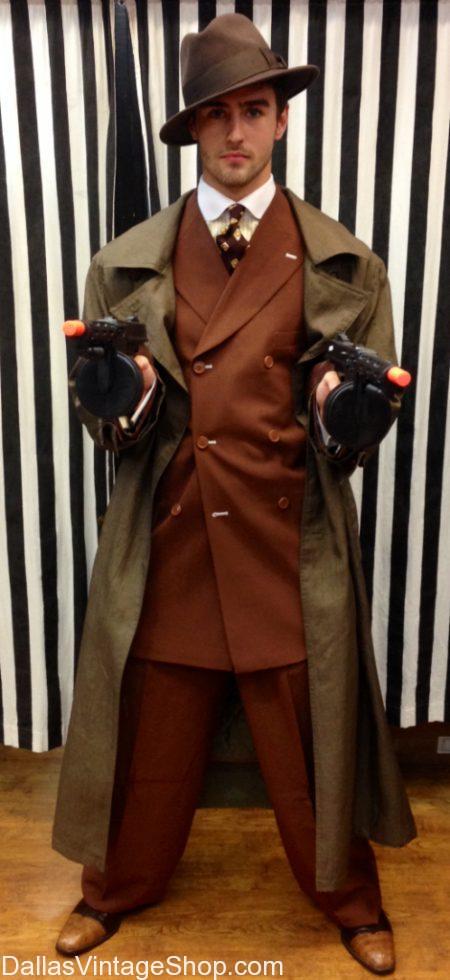This image captures a young white man in his twenties dressed as a 1940s-1950s gangster. He is wearing a loose-fitting, medium brown, double-breasted suit with baggy trousers, a white collared shirt, and a wide brown tie. Over the suit, he sports a dark tan trench coat. His ensemble is completed with a medium brown fedora, tilted jauntily to the side, and pointed brown leather shoes. He stands in a commanding pose, legs spread apart, holding a pair of black toy Tommy guns with orange tips to signify they are props. The backdrop features black and white vertical striped curtains, mimicking a dressing room. The photo, oriented vertically, shows him standing on a wooden floor. In the lower left corner of the image, the watermark "DallasVintageShop.com" is prominently displayed. The man gazes seriously at the camera, embodying a vintage gangster look reminiscent of historical gangsters like Al Capone.